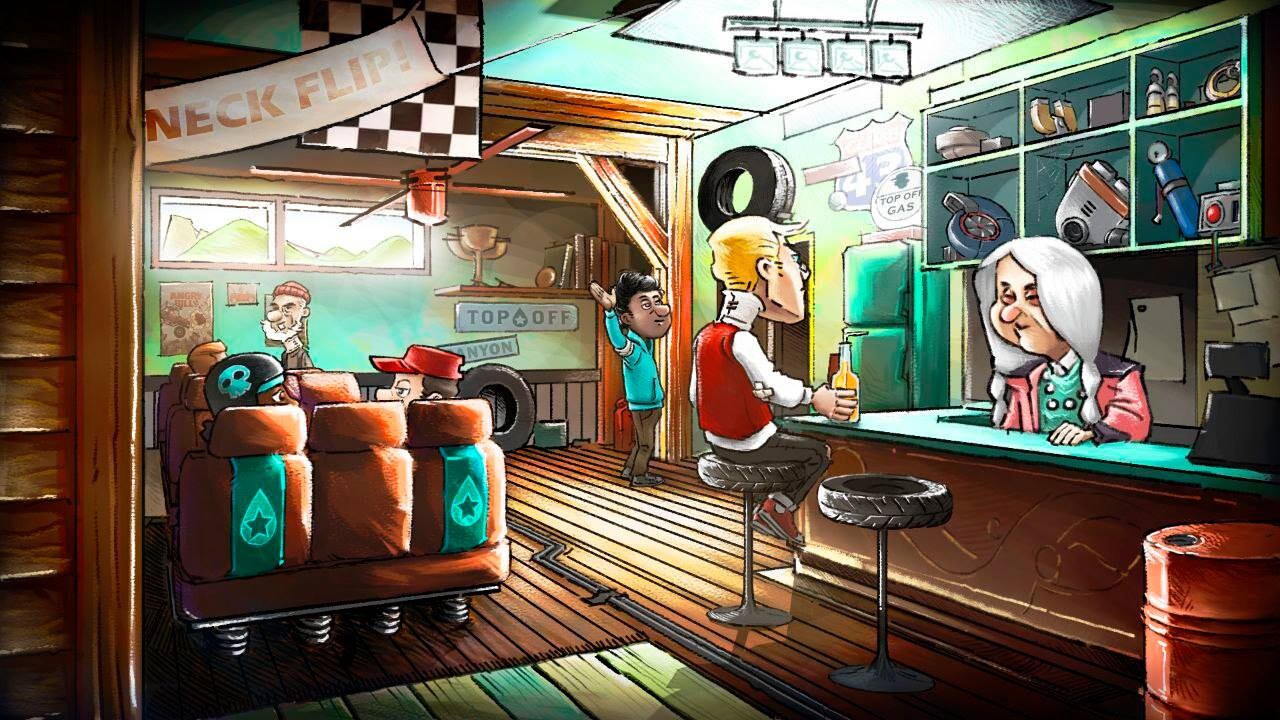This horizontally aligned rectangular cartoon image depicts a lively bar scene with an eclectic, salvaged theme. The focal point is an old woman with long, white hair styled in two braids, wearing a pink jacket over a light green shirt that matches the green countertop of the bar. She is leaning on the counter, while a blonde man in a white shirt with a red vest sits at the bar, his hand on a beer bottle, staring off into the distance. The bar's seating is creatively fashioned from vehicle parts, including tires and bus or van seats.

Above the bartender, shelves are lined with various knickknacks and pieces of equipment, alongside a cash register to her right. There is a red barrel at the bottom right of the scene. The wooden floor adds a rustic touch to the setting. In the background, a man in a teal long-sleeved top and tan pants raises his hand as if to wave or catch someone's attention. To the left, a couple sits in a booth engaged in conversation, under a banner that reads "Neck Flip." Behind this, another man stands by, seemingly inspecting posters on the wall. The overall cartoon style features exaggerated proportions, with the heads appearing larger than the body parts, contributing to the whimsical atmosphere of this uniquely styled bar.